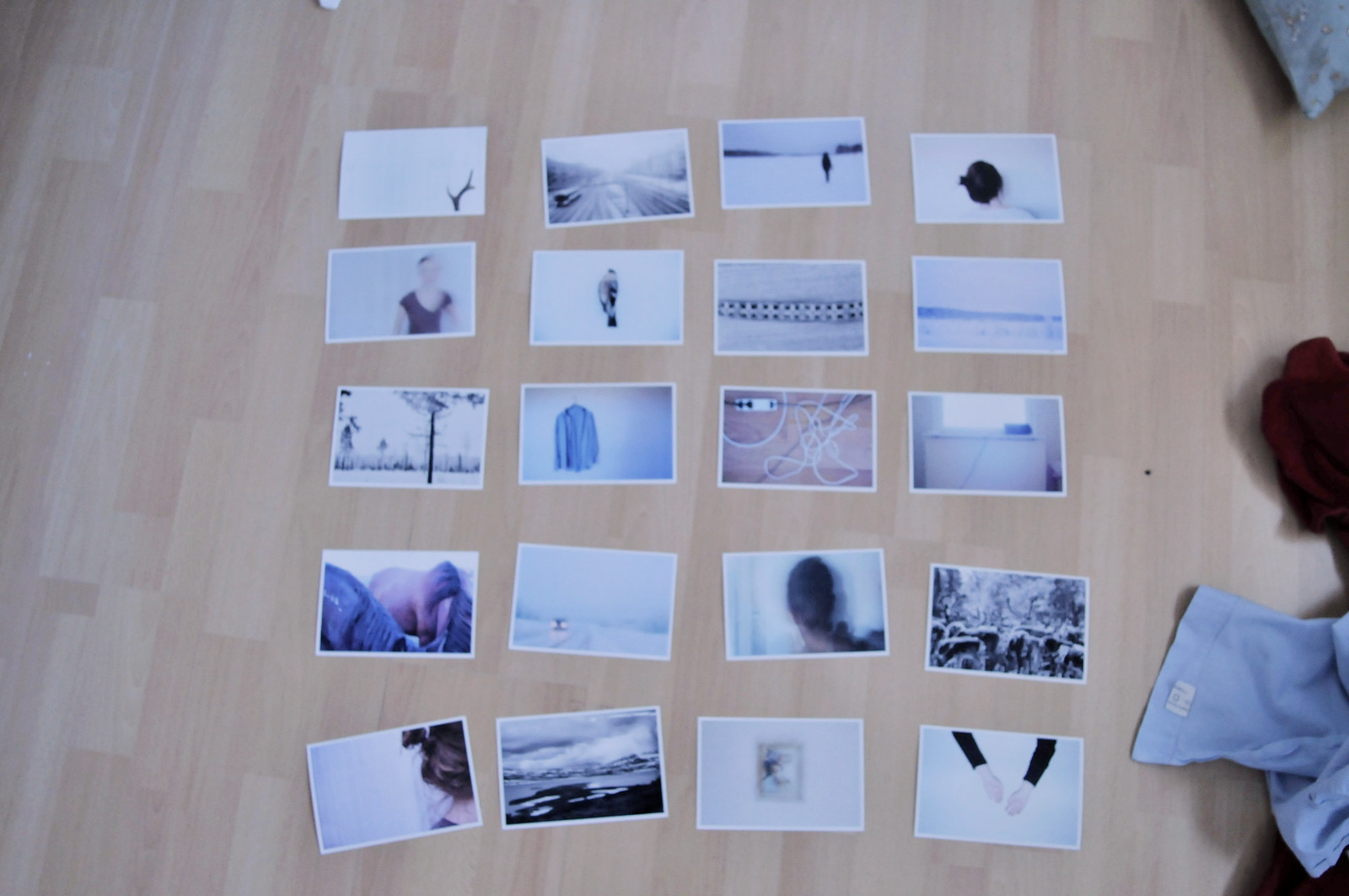The image depicts a lightly colored wooden floor with distinct planks, serving as the backdrop for an arranged display of twenty Polaroid photographs. The photos are meticulously laid out in five rows and four columns, each adorned with a white border. The photographs vary in subject matter, including abstract images, landscapes, people, and objects, such as a shirt and a person's arms. In the top right corner of the photo, the edge of a gray pillow can be seen peeking into the frame. Meanwhile, in the bottom right corner, there's a blue fabric with a white tag and a red piece of fabric, partially visible, suggesting the presence of clothes or laundry.